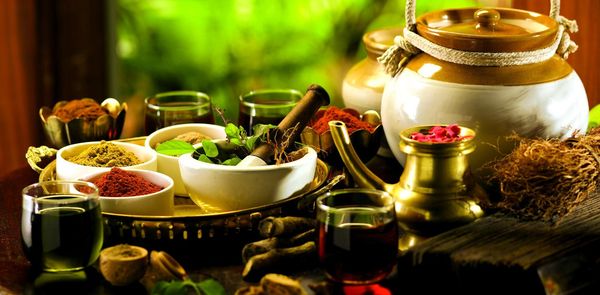The image depicts a carefully arranged scene, possibly on a dark wood or black kitchen or living room table, featuring a variety of culinary and decorative items. Dominating the right side of the image is a white teapot or sugar bowl with a brown top and lid. In front of this teapot is a golden holder containing rose petals and a short, squat glass that appears to hold either water or wine. Scattered across the table are four such glasses, adding a sense of symmetry.

Towards the left side, a prominent golden serving tray is laden with four white bowls. Three of these bowls contain different spices—one with a red spice and two with brown spices—while the fourth holds green leaves and a mortar and pestle, suggesting ingredients ready to be ground. Additional items include glasses with varied liquids, possibly tea or oils, and a golden container with a long spout, probably for dispensing oil.

The background is artfully blurred but reveals hints of a wooden wall and a window with greenery, adding to the warm, homely atmosphere. Among other objects are a bundle of grass-like substance tied with a string, a green leaf, and a little wooden container, all contributing to the rich, textured composition of the scene. The overall arrangement evokes a sense of cozy domesticity, intricately tied with culinary artistry.